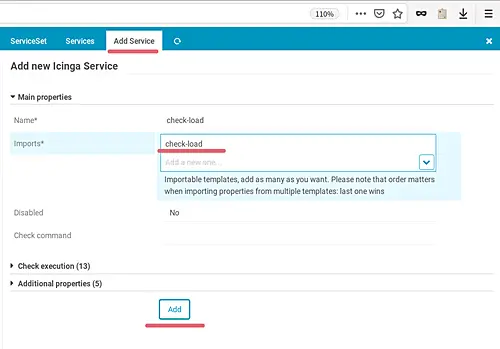This digital image showcases a detailed interface for managing services. At the top, there is a header displaying "110%." Under this header, you can find options like "Service Set," "Services," and an "Add a Service" button, accompanied by a refresh button. A close button marked with an 'X' is also present. The interface prominently features an "Add New" section, specifically for adding a new "Instica Service." 

In the "Main Properties" section, you can input the service's name and manage imports, with "Check Load" field appearing twice, once as a text and a second time in a drop-down menu. Below this, there is a section for "Importable Templates," where you can add multiple templates with a note emphasizing that order matters — the last template imported will take precedence. 

On the left side of the interface, there is an option labeled "Disable" with a corresponding "No" on the right side. Below the drop-down, in gray font, is "Check Command." Further down, in bold black font, is "Check Execution" with a "(13)" indicator. Below that, another section labeled "Additional Properties" also includes a "(5)" indicator. 

At the bottom of the interface, a blue and white "Add" button is flanked by a prominent red bar beneath it.